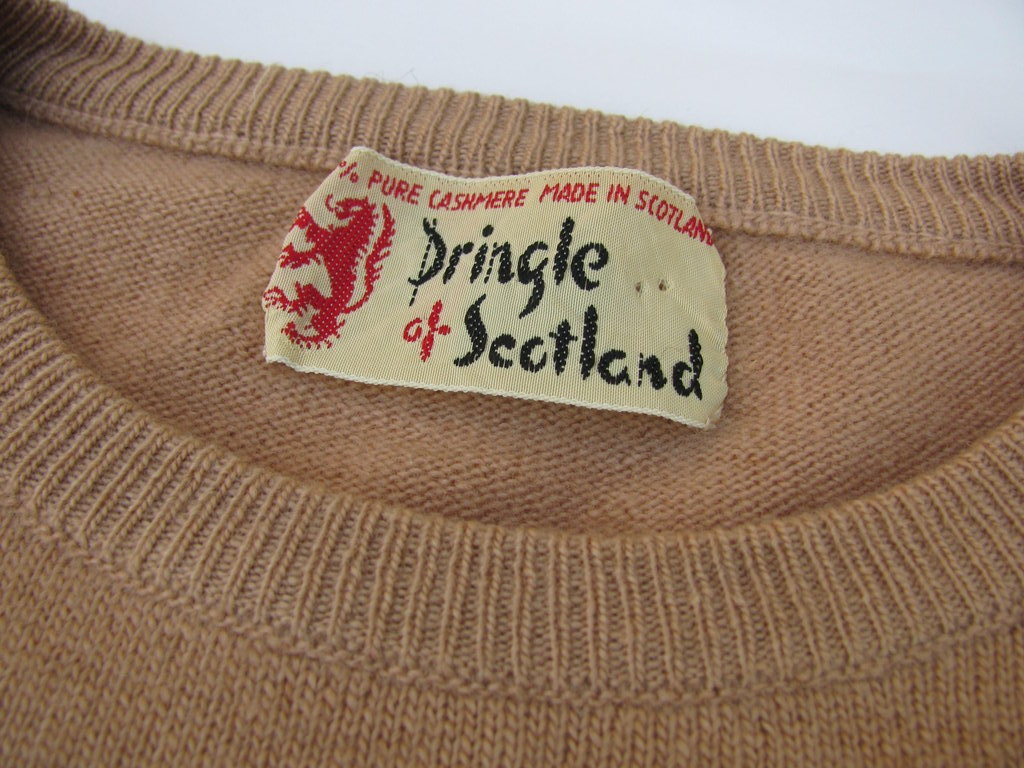This close-up photograph showcases the intricate details of a tan-colored cashmere sweater, particularly emphasizing its neck area and label. The sweater, made of fine fabric, features visible stitching around the elastic neckline. A significant portion of the image focuses on the rectangular tag, which is a cream color. Prominently displayed on the left side of the tag is a detailed red logo depicting a mythical creature resembling a dragon or lion, complete with four arms, a long tail, and a protruding red tongue. The text on the tag reads "Pure Cashmere Made in Scotland" in red text at the top, followed by "Pringle" in black, "of" in red, and "Scotland" in black. Additionally, there are two small holes punched above the "N" in "Scotland," likely from a pin or attachment. The background of the image is a light blue-white color, which further accentuates the focused details of the sweater and its label.